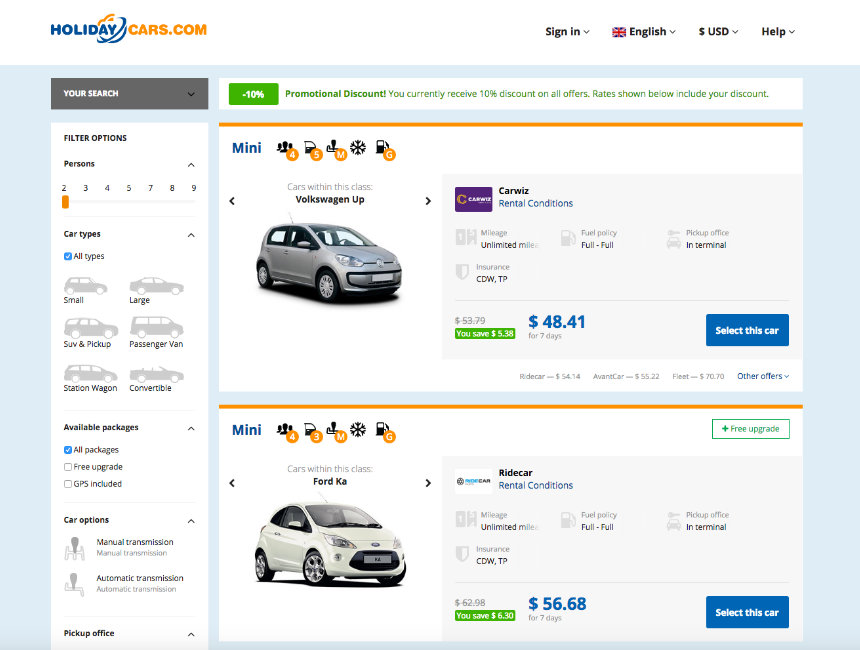The image is a cropped screenshot of the holidaycars.com webpage, presented against a white background. The top left features the holidaycars.com logo, and to the far right of it, there is a "Sign In" button accompanied by a right-facing arrow for category expansion. To its immediate right is the word "English" with a British flag icon next to it, and a downward-facing arrow indicating a drop-down menu. Further right, it displays "US Dollars" with another downward arrow, and finally, a "Help" button.

On the left side of the page at the top, a small bar labeled "Your Search" in white letters is displayed. Directly below this bar is a long vertical white section featuring filter options. The first filter reads "Persons" in bold black letters, with a slider bar beneath it set to 2. Next is "Car Types" also in bold black letters, with the option "All Types" in smaller black font and a selected checkbox beside it.

Below this, the "Available Packages" filter is presented with three options, of which "All Packages" is currently selected. Following that are "Car Options," providing choices for manual and automatic transmissions, though neither has been selected.

The left side of the screenshot also lists two vehicle options. The first is from CarWiz, and the second is from RideCar, both indicated to be small economy cars. Each listing includes the price, a thumbnail image of the car, and a blue button labeled "Select This Car" on the bottom right.